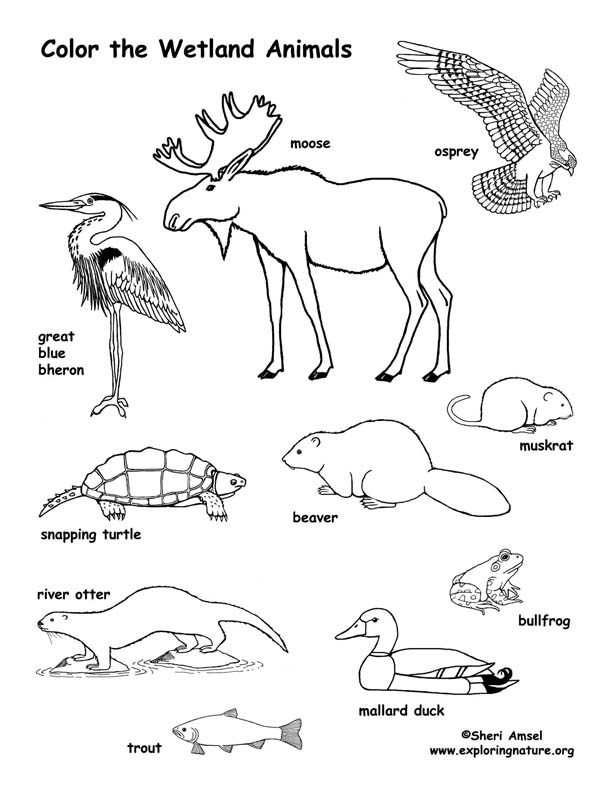This is a detailed, black-and-white illustrated coloring page titled "Color the Wetland Animals" designed by Sherry Amsel, available on www.exploringnature.org. The illustration displays a variety of wetland creatures arranged from left to right, including a great blue heron, a moose, and an osprey in mid-flight. Below them, a snapping turtle, beaver, muskrat, river otter, mallard duck, bullfrog, and a trout are depicted, most in broadside view. The animals are drawn as detailed sketches, with minimal background and no color, allowing for personal coloring. Noticeably, while most animals face left, the osprey, muskrat, snapping turtle, and bullfrog face different directions, adding visual interest. The illustration ends with the artist’s name and copyright information at the bottom of the page.